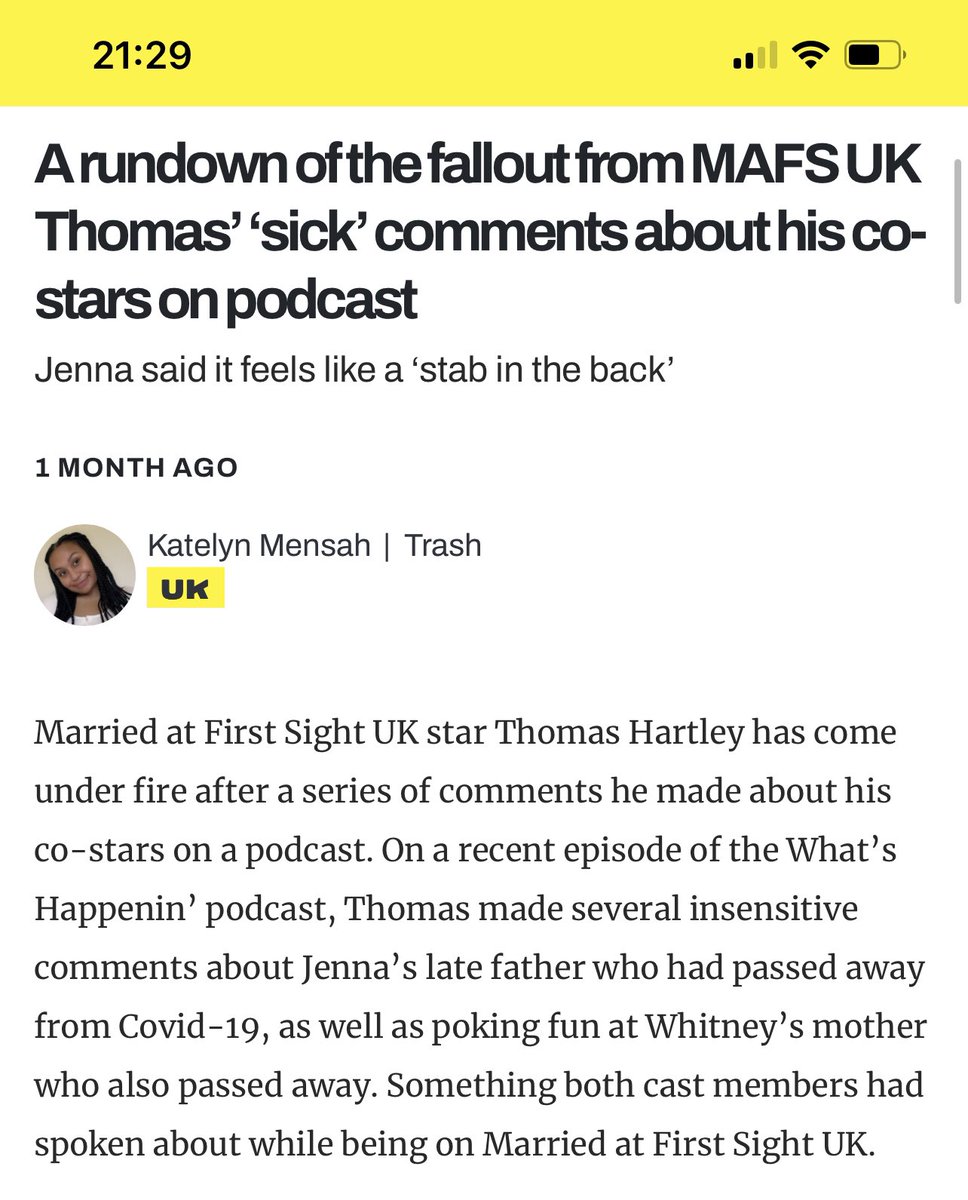This is a detailed screenshot from a cell phone, displaying an article under a yellow banner at the top which shows the time as 21:29, alongside icons for service bars, Wi-Fi, and battery status on the upper right. The headline reads: "A Rundown of the Fallout from MAFS UK Thomas's Sick Comments About His Co-Stars on a Podcast. Jenna Said It Feels Like a Stab in the Back." This article is timestamped as from one month ago. Beneath the headline is a circular photograph of a young black woman with braided hair, tilting her head to the left. Next to her photo is the name "Caitlin Mensah" and the word "trash" following a slash. Additionally, there is a small yellow rectangle below her name that says "UK" in black letters. The article begins with, "Married at First Sight UK star Thomas Hartley has come under fire after a series of comments he made about his co-stars on a podcast. On a recent episode of the What's Happening podcast, Thomas made several insensitive comments about Jenna's late father, who had passed away from COVID-19, as well as poking fun at Whitney's mother, who also passed away—subjects both cast members had discussed while on Married at First Sight UK."